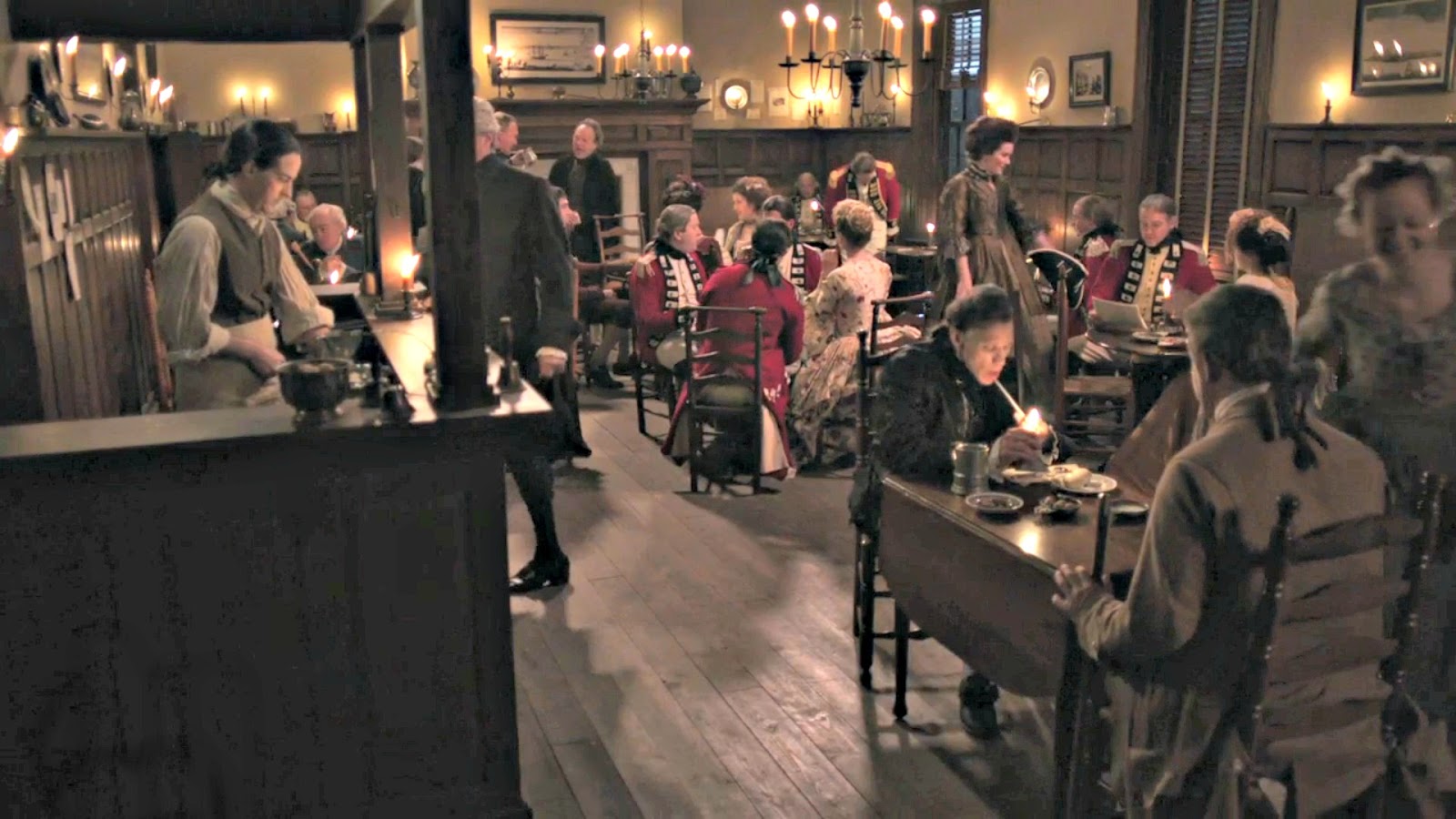This meticulously detailed image portrays a vivid recreation of an 18th-century American tavern scene, likely reminiscent of the American Revolution era. The foreground and background are filled with men dressed in red coat uniforms, complete with white shirts, patterned sashes or scarves, and distinctive wigs or hair pulled back into ponytails. These "redcoats," representing British soldiers, are seated at several round and oblong tables, and one man at the front is seen smoking a cigar or pipe.

Central to the image is the indoor tavern setting, characterized by its dim, candlelit ambiance. Numerous candles adorn the walls and a grand chandelier, casting a warm glow without any sign of dripping wax. On the right side of the image are windows fitted with blinds, adding to the authentic period detail. 

On the left, a barkeep stands behind the bar, sporting black hair tied back into a bun. He dons a brown vest over a long-sleeved gray shirt, the sleeves of which are puffy or rolled up. In this bustling establishment, another figure—dressed entirely in black—stands at the bar, though his face is obscured.

Among the patrons is a genteel lady in a modest, long dress, her arms covered past the elbows, signifying the fashion of the time. Another woman in the foreground wears a white bonnet, further grounding the scene in its historical context.

The tavern, furnished with wooden tables and an array of period-appropriate details, including a prominent large fireplace at the back of the room, offers an immersive glimpse into a bygone American era, captured in strikingly lifelike colors and high detail.